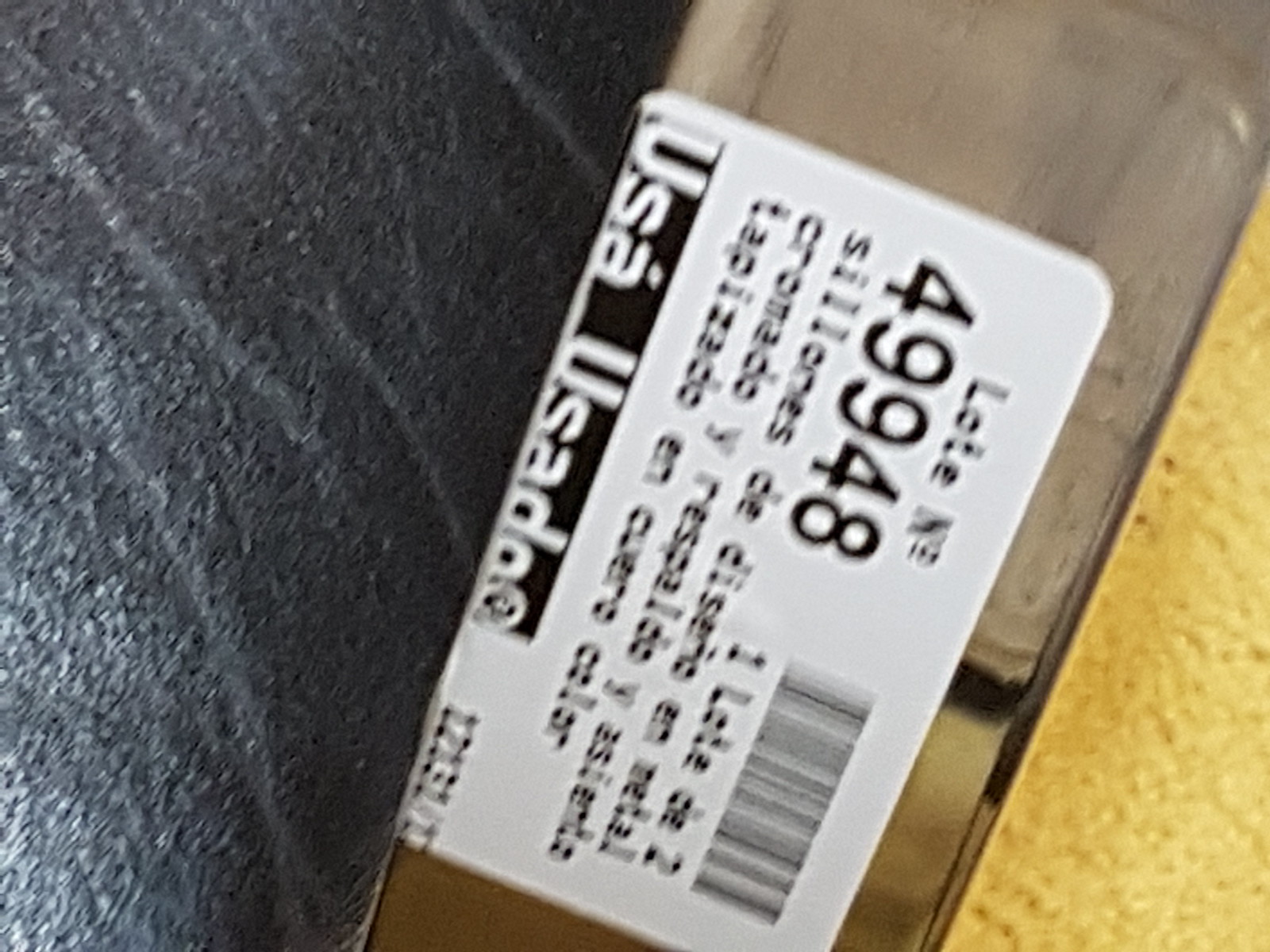This square-shaped image features a silver-colored item at its center, adorned with a white sticker. The sticker is positioned sideways and contains black print. Notably, a barcode in black and white is located at the bottom right of the sticker, while the top right corner displays the text "L-O-T-E." The left side of the image is completely filled with a solid black color, and the bottom right corner features a block of yellow, creating a stark contrast with the monochromatic tones of the sticker and the silver item.